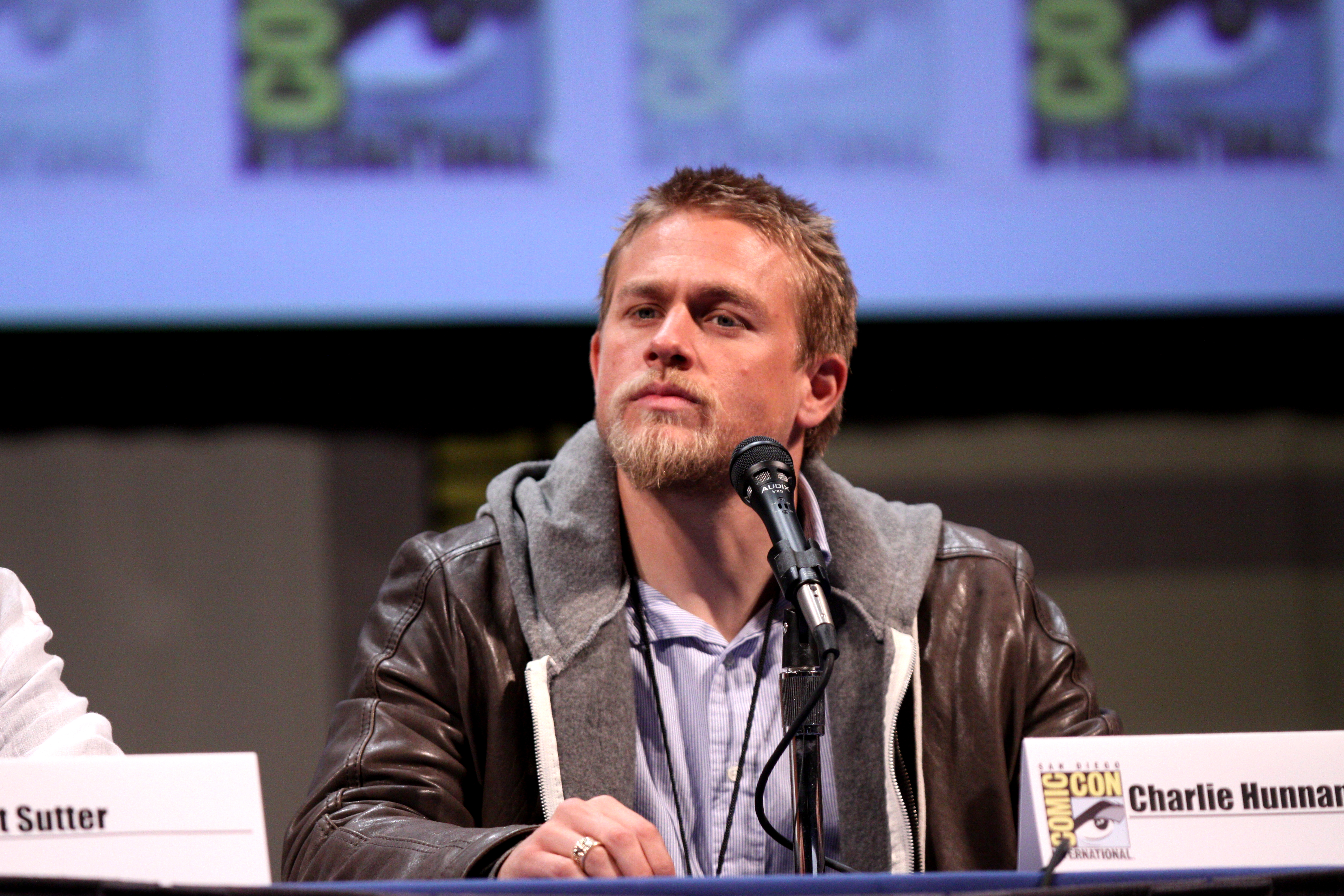The image depicts a man named Charlie Hunan, seated at a podium on a dais. He is wearing a brown leather jacket layered over a zip-up hoodie and a gray button-up shirt. Charlie has blonde hair and sports a beard and mustache. He is in the middle of a presentation at Comic-Con, as indicated by the Comic-Con logo to the left of his name placard, which partially reads "Charlie Hunan." In front of him, there is a black microphone. In the background of the indoor setting, the wall transitions from a purple color to brown halfway down. To his left, another name tag partially reads "Sutter" next to a person in a white shirt. Charlie appears to be engaged and focused as he looks out at the audience.